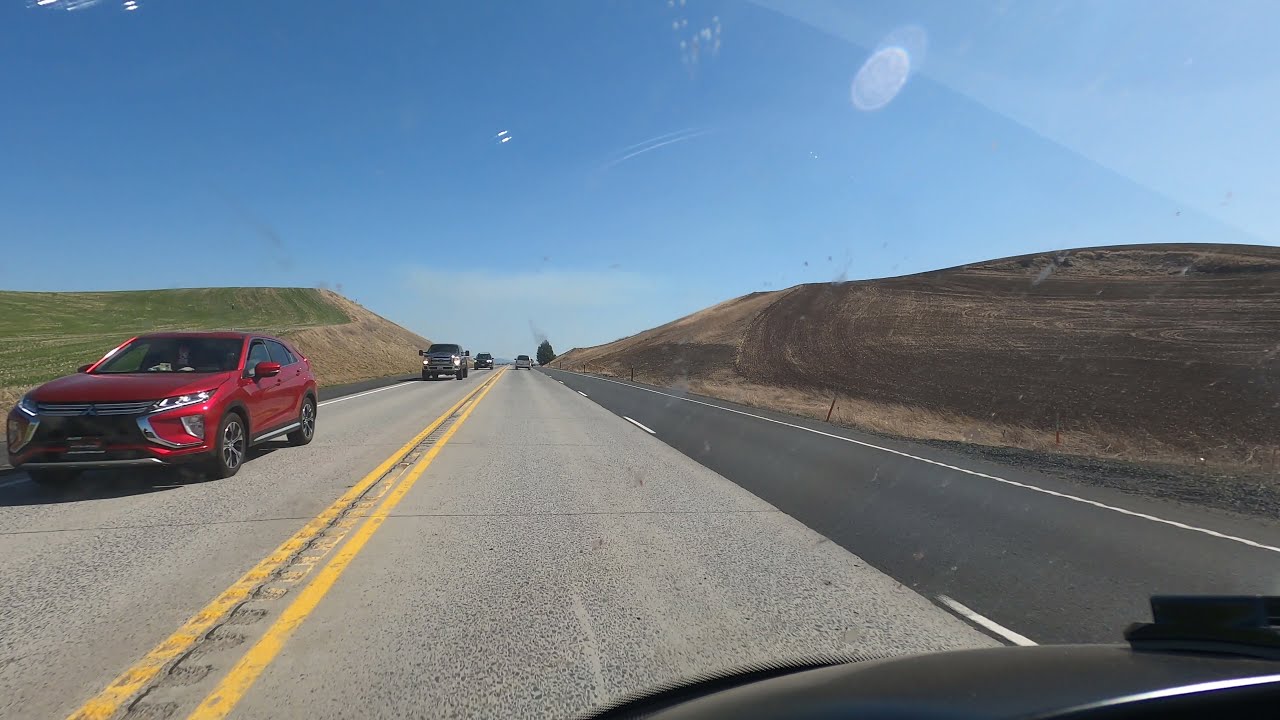The image depicts a rural two-lane highway under a cloudless, vivid blue sky. The road is paved with light-worn gray asphalt, and a double yellow line separates the two opposing lanes of traffic. There is a darker, newer black lane on the far right, marked by a white edge line. Various dirt treads on the right shoulder indicate frequent vehicular use off the main road. On the left of the highway, a grassy hill rises gently, while a similar hill on the right side shows signs of dirt. 

Foreground views suggest that the picture is being taken from inside a black car, peering over a dark dashboard. Several vehicles are on the two-lane road, including a conspicuous red four-door car in the left oncoming lane, a black truck, and a possible black SUV. In front of the photographer's car, a silver van can be spotted. The overall scene is bathed in bright, sunny weather, implying it might be quite warm outside, akin to a rural stretch of the highway one could encounter in Illinois, nestled between larger and smaller cities.